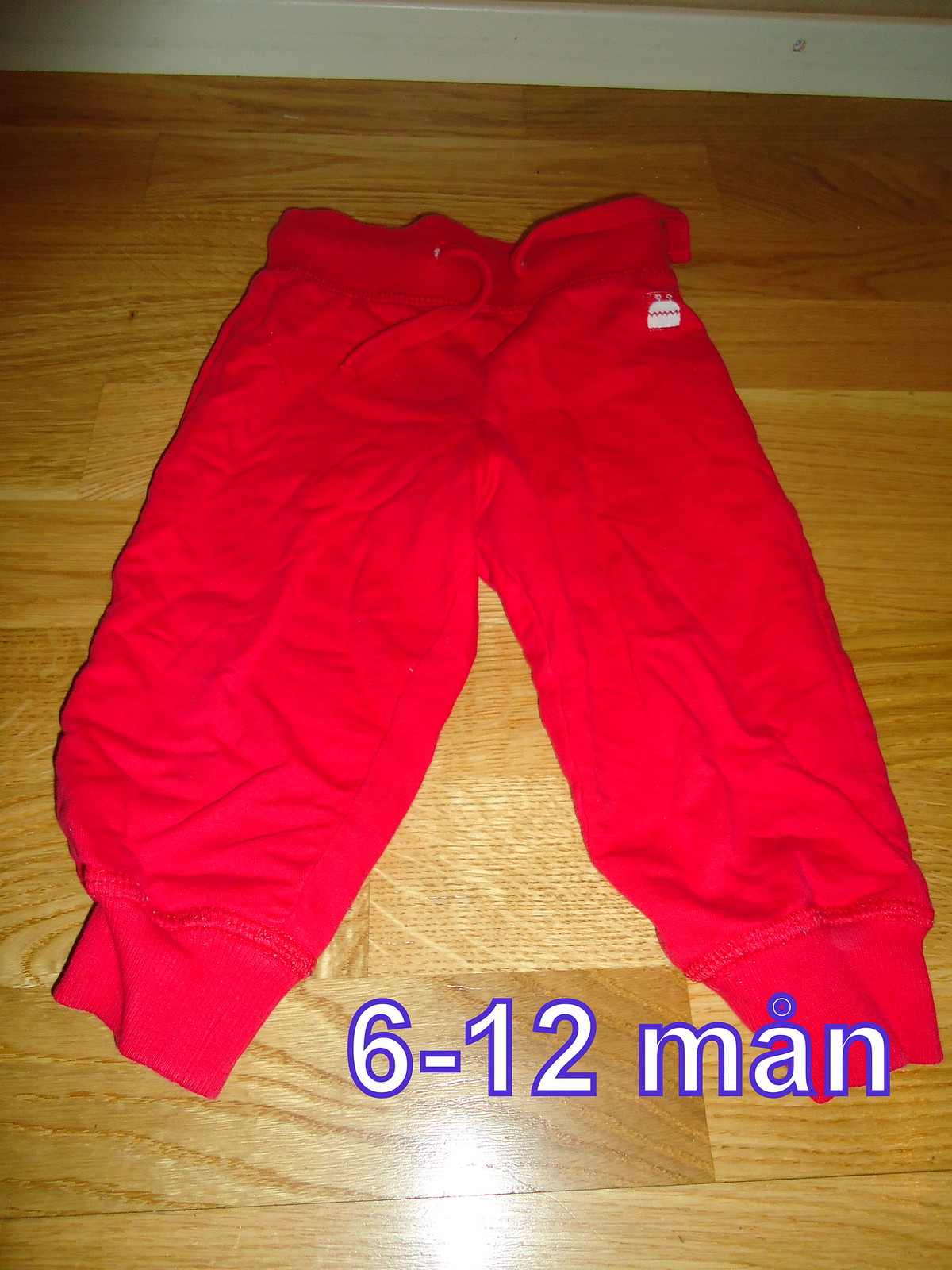This image features a pair of red exercise pants, most likely sweatpants, laid flat on a hardwood floor. The sweatpants are positioned with their legs slightly apart and are noticeably wrinkled, suggesting they haven't been ironed. At the waist, there are two red tassels for the drawstring closure. A distinctive white logo, which appears to resemble a stylized face with eye stalks or possibly a cracked eggshell with a rectangular base, is situated near the left hip. Additionally, there’s text at the bottom of the pants reading "6-12 man," with a unique circle above the 'A' in "man." The photo is taken with the pants on a wooden laminate floor, visible with reflection possibly due to the use of a flash. The baseboard molding along the wall is white, contrasting with the floor.